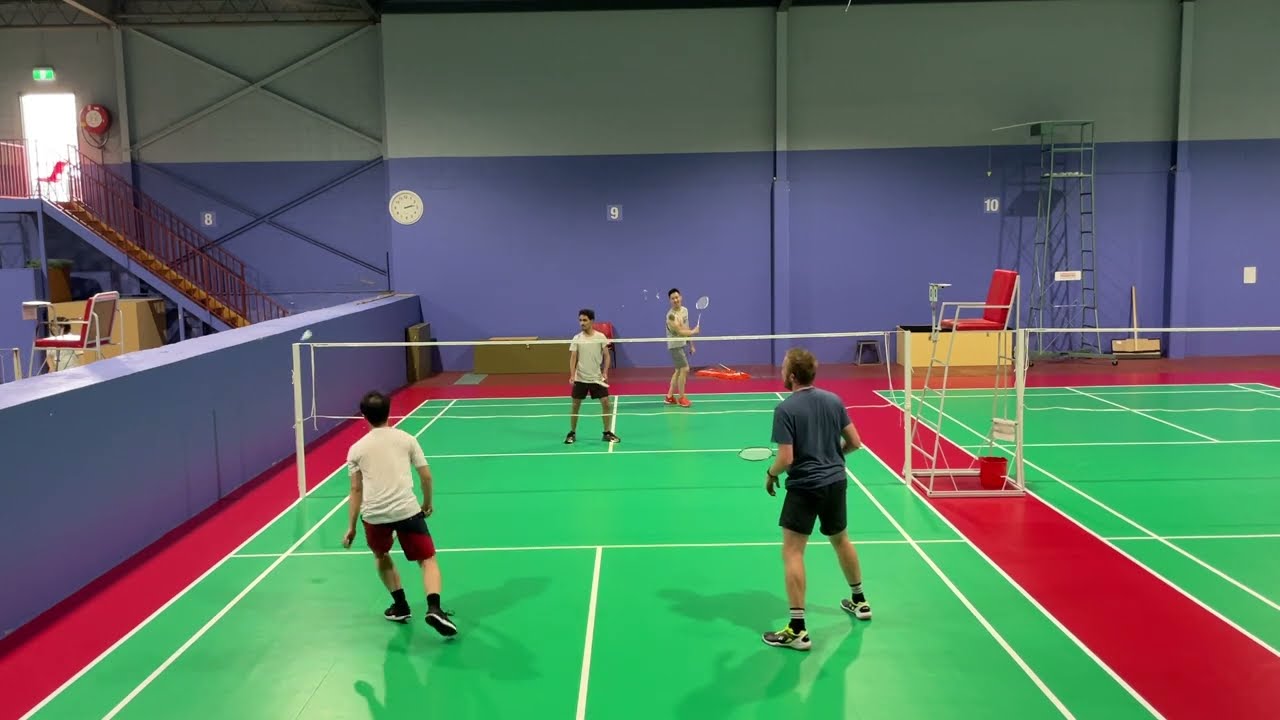The photograph captures an indoor badminton facility characterized by its industrial aesthetic, featuring a vivid array of colors and structural elements. The spacious indoor area houses two adjacent green badminton courts marked with precise white lines for player positioning. The main focus is on the court in the center where four men are actively engaged in a game, with two players positioned at the front and two at the back, each holding their badminton rackets. A distinctive net spans the middle of the active court, and adjacent to it is an elevated red referee chair perched on a square metal frame, resembling a lifeguard chair, ensuring a clear view of the game. The surrounding floor area outside the courts is a muted red, contrasting with the court's green. The facility's walls exhibit a dual-tone design: the lower half is painted purple or light blue, and the upper half showcases a green or white hue. Additional structural features include stairs leading up to a door in the top left corner and visible steel framing that supports the high ceiling, emphasizing the warehouse-like atmosphere of the venue.